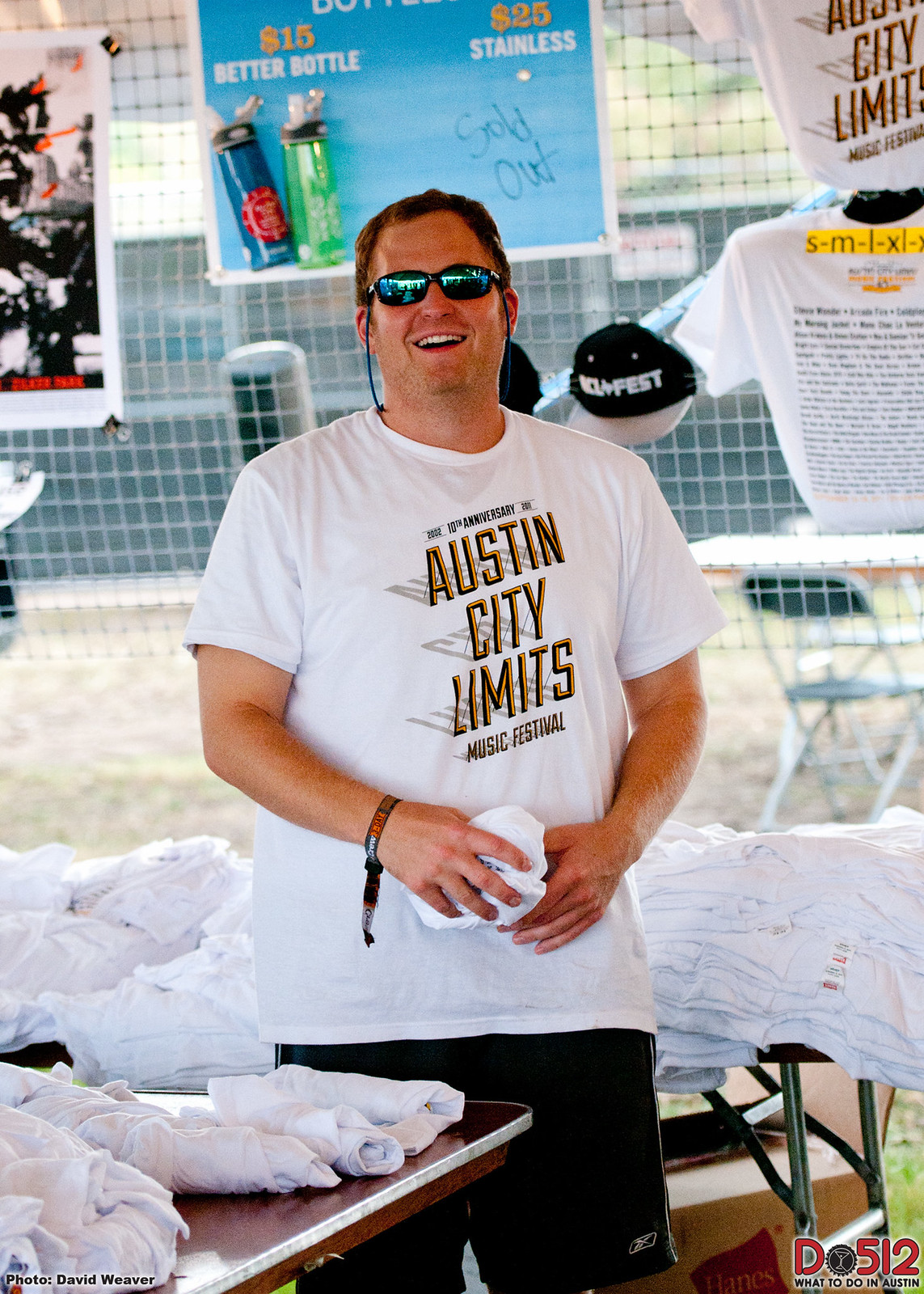This image captures a cheerful man participating in what seems to be a music festival, likely the Austin City Limits Music Festival, given his attire. Dressed in a white short-sleeved t-shirt emblazoned with "Austin City Limits Music Festival," black shorts, and mirrored blue sunglasses, the man stands confidently beside two tables loaded with t-shirts, some rolled up and others laid flat in large piles. He has a black wristband with red and white lettering and is holding a t-shirt in his hand. The setting appears to be an outdoor tent with a netted, mesh-like structure in the background, adorned with additional merchandise, including baseball caps, various t-shirts, and water bottles. Signs attached to the mesh indicate prices for these items, such as "Better Bottle, $15, Stainless, $25," and a "sold out" notice can also be seen. A Hanes t-shirt box is visible under one of the tables, further suggesting that the man is vending apparel at this event. The scene is bright and vibrant, capturing the bustling atmosphere of a lively festival.